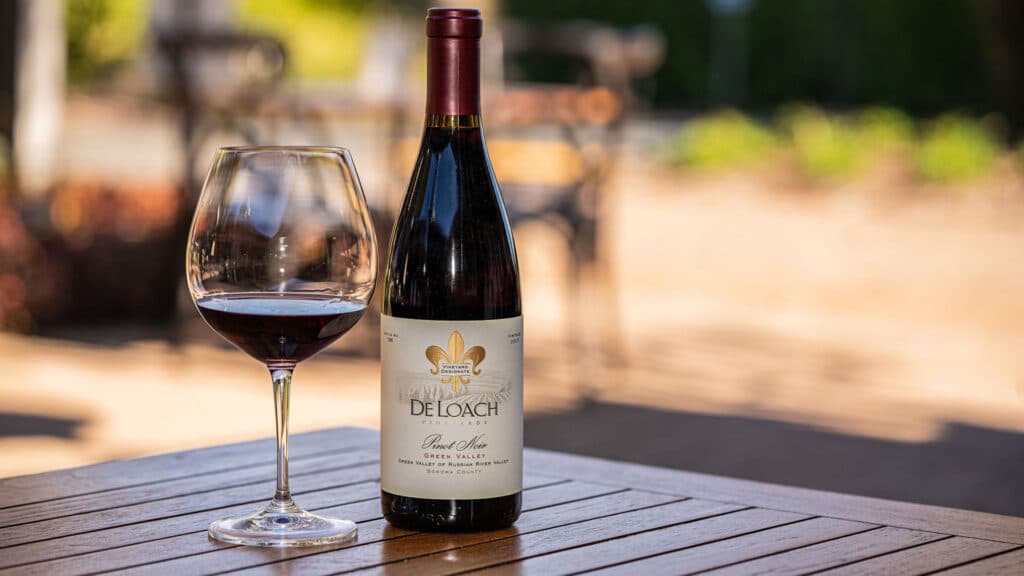The image is a detailed color photograph taken outdoors, likely at the Deloche Vineyards in the Green Valley of the Russian River Valley, Sonoma County, California. The primary subjects are a bottle of vintage 2017 Deloche Pinot Noir and a long-stemmed red wine glass with a small pour of the wine. The bottle prominently displays its red and white label, identifying it as bottle number 156. The scene is set on a wooden table with long slots, and the glass beside the bottle is notably untouched and pristine, suggesting it is ready to be enjoyed. The background is blurred but reveals hints of a sunny, warm atmosphere with light filtering through, possibly indicating other tables, chairs, and some greenery in the distance. The inviting ambiance highlights the wine and glass, making them the focal points of this inviting, serene scene.